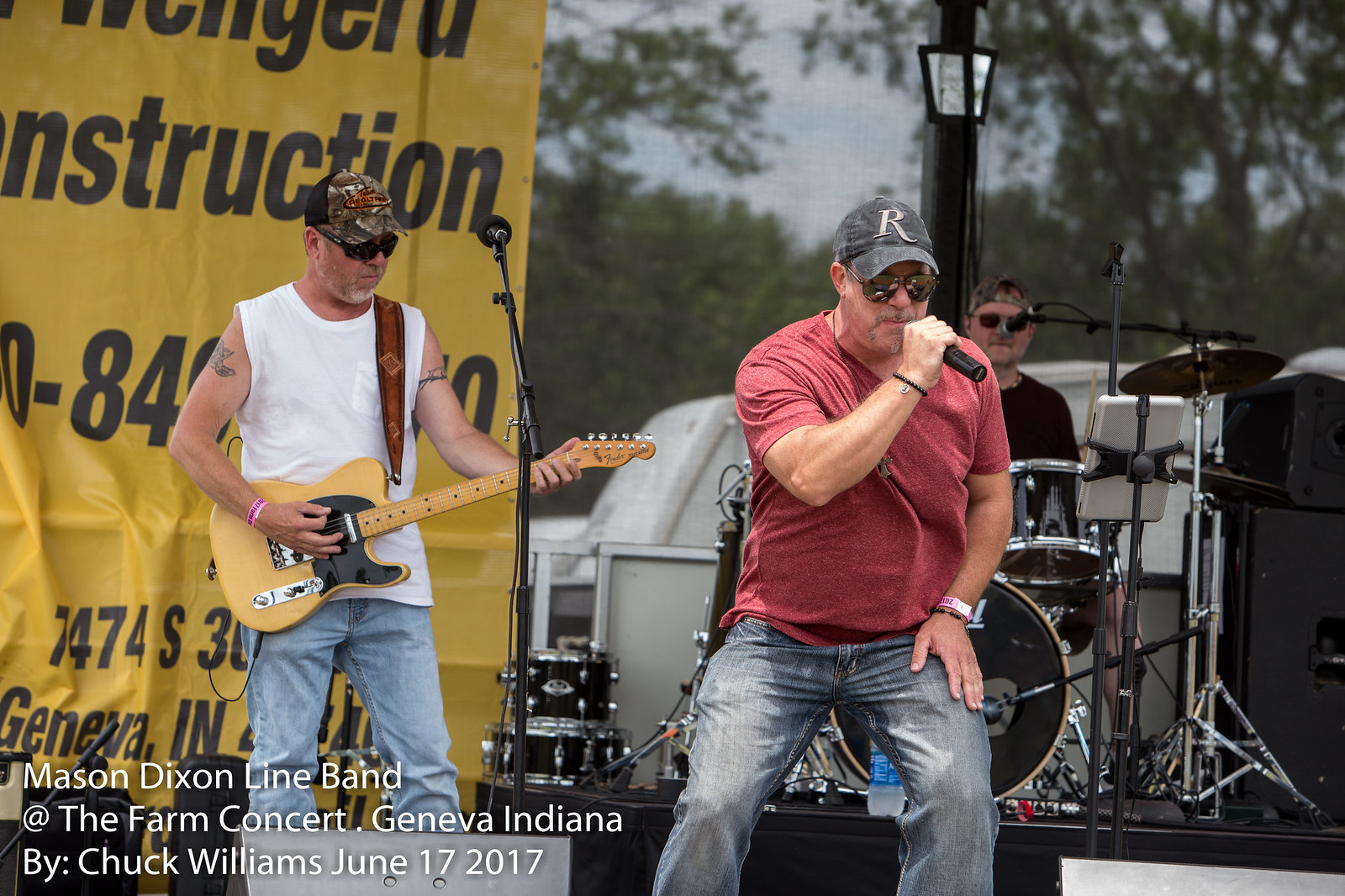This detailed photograph captures the Mason Dixon Line Band performing at The Farm Concert in Geneva, Indiana, on June 17, 2017. The image, credited to Chuck Williams, features three band members against an outdoor backdrop of trees and an overcast sky. In the foreground, the lead singer, wearing a red V-neck T-shirt, faded blue jeans, and a blue hat with a stylized "R," is holding a microphone in his right hand, partially crouched with aviator sunglasses on. To his left, the guitar player, clad in a sleeveless white shirt, blue jeans, and a camo hat, strums an electric guitar with a black pickguard. He sports sunglasses, a gray goatee, and visible tattoos on his shoulders. Behind them sits the drummer, dressed in a dark shirt and headband, playing a black drum set, with a microphone positioned for him to also sing. A yellow banner with the barely visible text "construction" and contact information, along with a light pole, further accents the setting. The lower-left corner of the photo features the caption: "Mason Dixon Line Band at The Farm Concert, Geneva, Indiana, by Chuck Williams, June 17, 2017."